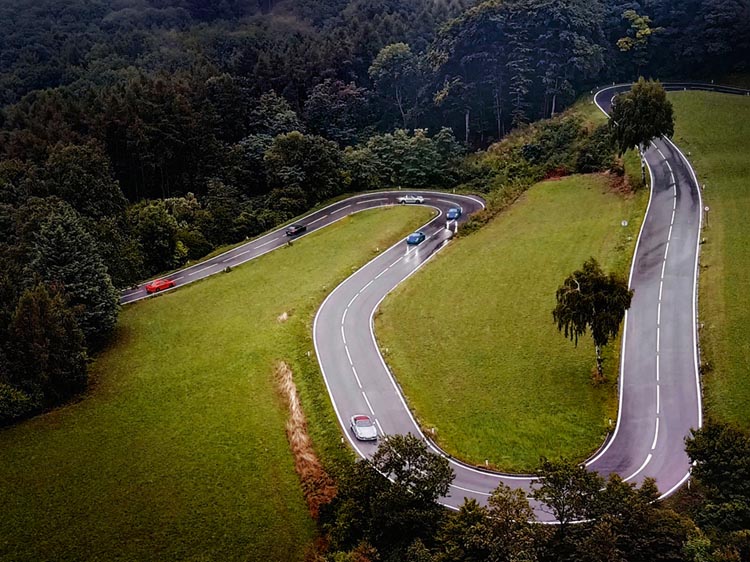This aerial photograph captures a vividly green landscape dominated by a winding road. The road, appearing wet as if it's been raining, snakes through large grassy fields, creating a series of switchbacks as it ascends a slope. The scene suggests a mountainous region with lush greenery. In the upper left corner and extending across the top of the image, a dense forest of dark green trees frames the landscape, contrasting with the vibrant green fields below. Scattered within these fields are isolated trees, adding texture to the scene. The road itself is dotted with six cars, including a couple of blue ones, a white convertible, a black car, a silver car, and a red car, all traveling uphill from the left to the right, indicating a right-hand driving system. The intricate layout of zigzagging roads and the varied shades of green paint a tranquil yet dynamic scene, giving the impression of a tropical, mountainous area, though its exact location remains unspecified.